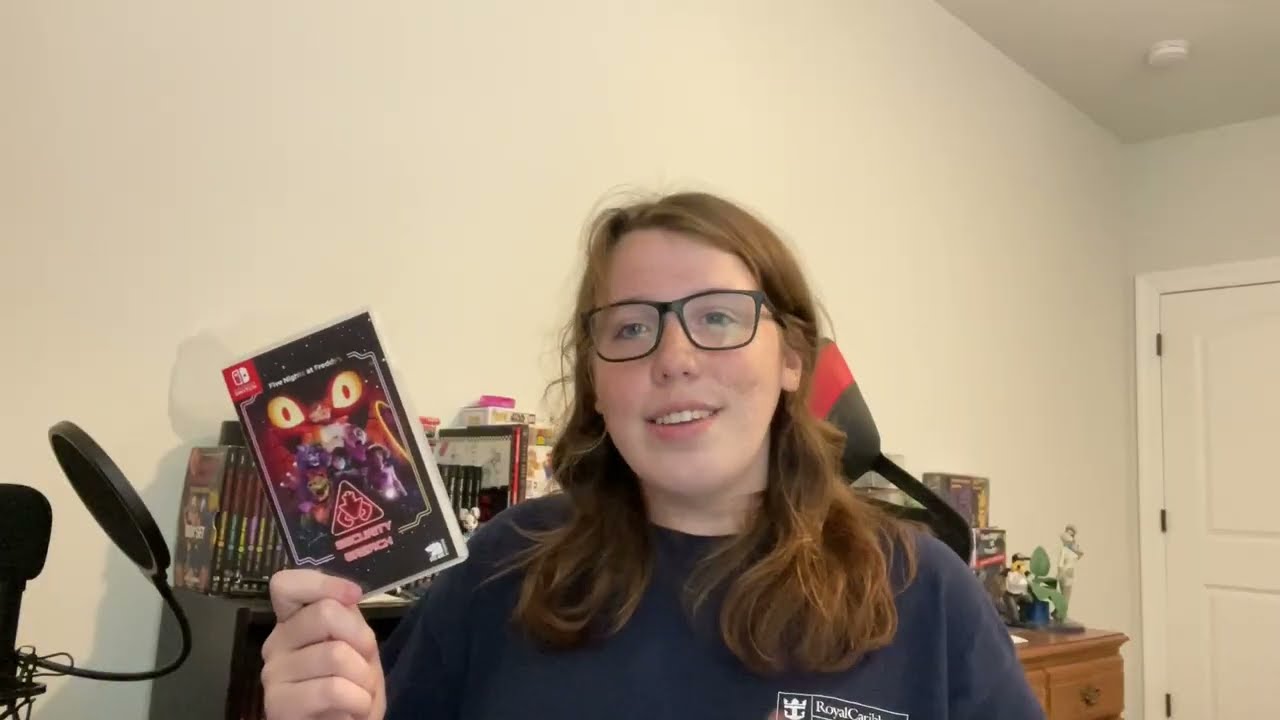The image captures a late teenage or early 20s young woman seated in a black and red gaming chair, likely in her bedroom. She has long, auburn hair that falls below her shoulders, accented with dark-rimmed glasses, and faint freckles. She wears a navy blue t-shirt with a Royal Caribbean Cruises logo on the left breast. The woman is smiling slightly as she looks into the camera, holding up a rectangular Nintendo Switch game package for "Five Nights at Freddy's: Security Breach," identifiable by its cover featuring large yellow eyes and eerie characters.

She appears to be mid-sentence or speaking, possibly part of a video or stream, as indicated by her professional microphone positioned just to the left of the frame. Behind her, the room features white walls with no decorations, a desk cluttered with multiple books that resemble manga or DVDs, and a small sculpture. A dresser and bookshelf are also visible, alongside a door on the perpendicular wall near the photo's right edge. Additionally, a smoke alarm is mounted on the ceiling. The overall scene suggests a casual, cozy residential setting.